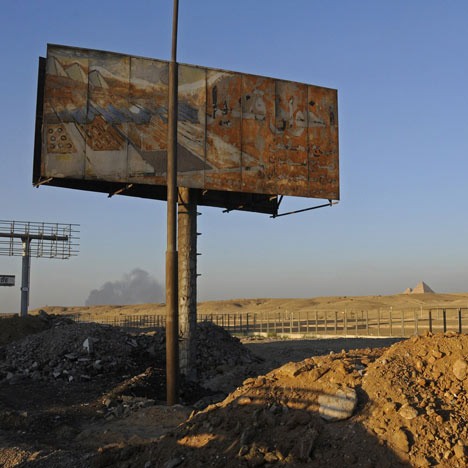The image portrays a desolate outdoor scene dominated by a relic of the past—a severely weathered and rusted billboard at the center, standing sentinel among mounds of reddish-brown dirt and scattered rocks. Although the image on the billboard is now indiscernible, hints of vibrant graffiti with reds, yellows, and whites hint at its former message. Nearby, a tall light pole ascends towards a pristine, cloudless blue sky, with a large antenna stretching groundward, hinting at forgotten communication. The setting appears to be a construction zone devoid of buildings, where earth has been dug up and abandoned. To the left of the billboard and near its rear, a dilapidated wood plank fence or corral-type structure barely stands. Far in the distance, the barren landscape slopes into rolling hills and a diminutive pyramid-like peak, accentuating the scene's sense of arid vastness.